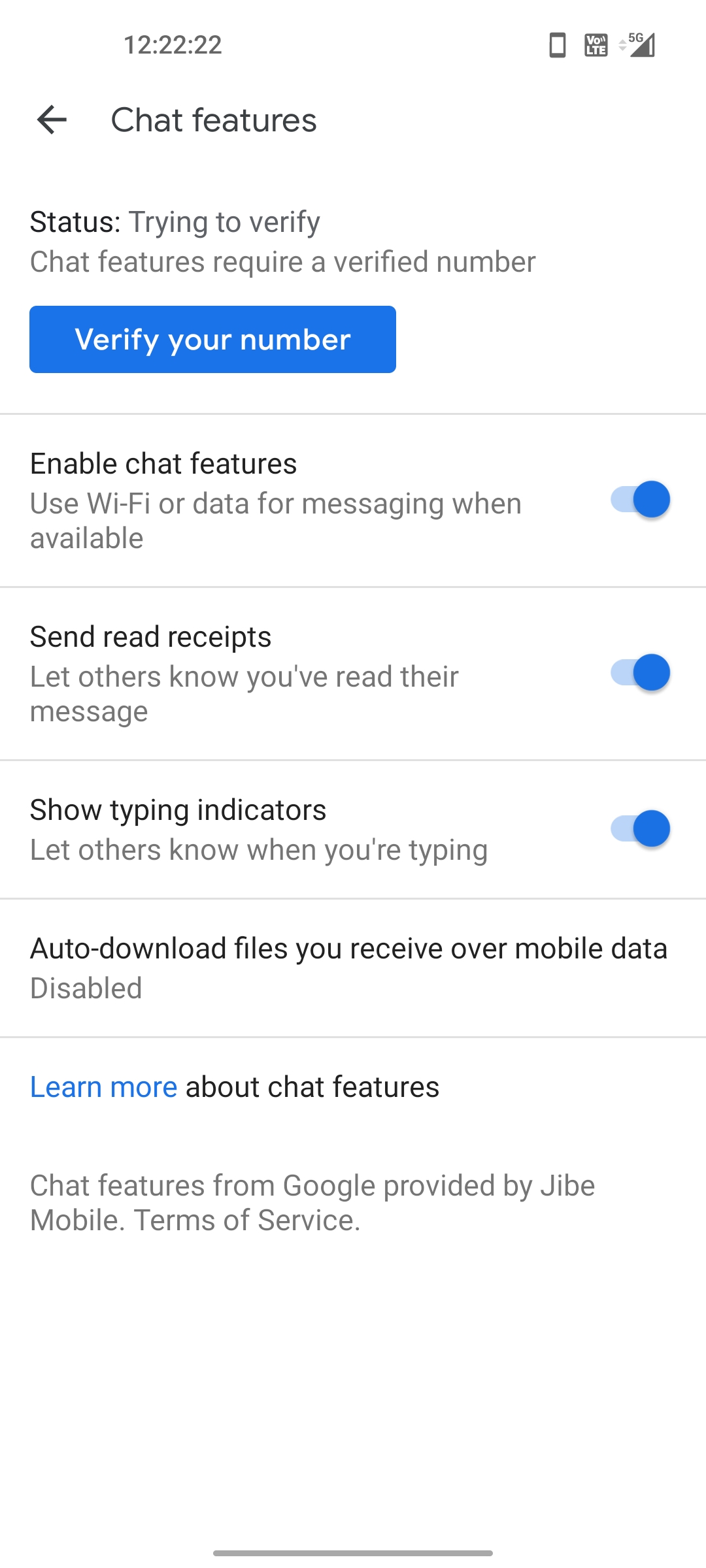This screenshot appears to be from the settings screen of a tablet or smartphone, likely taken at 12:22:22, possibly in military time. In the top right corner, various status icons can be seen, including a phone symbol with a black bezel on both the top and bottom, adjacent to a black square displaying "VO...LTE" in white text. Additionally, gray up and down arrows are present, alongside nearly full cell signal bars under the label "5G".

The main content of the image focuses on the "Chat Features" settings screen. On the left, a black arrow points back to the previous menu, and the heading "Chat Features" is prominently displayed in bold black text. Below that, the "Status" is indicated in bold black, followed by ellipses and the message "Trying to verify" in either gray or black text. Adjacent to it, a gray message states, "Chat features require a verification number." A dark blue button with white text prompts users to "Verify your number."

In a new section labeled "Enable chat features," bold black text explains that Wi-Fi or data can be used for messaging when available. A slider with a cyan blue background and a dark blue circle at the front indicates this feature is turned on. Similar settings include "Send read receipts," which allows others to know when you've read their message, and "Show typing indicators," which lets others know when you are typing; both options have their respective explanations in gray text and are enabled with sliders.

The subsequent sections lack sliders. "Auto download files you receive over mobile data" appears in black text and is marked as "Disabled" in gray text. A hyperlinked blue text states "Learn more about chat features." Lastly, the footer notes "Chat features from Google provided by Jibe Mobile. Terms of service," concluding with a small gray oval for navigation and exit functionality at the bottom of the screen.